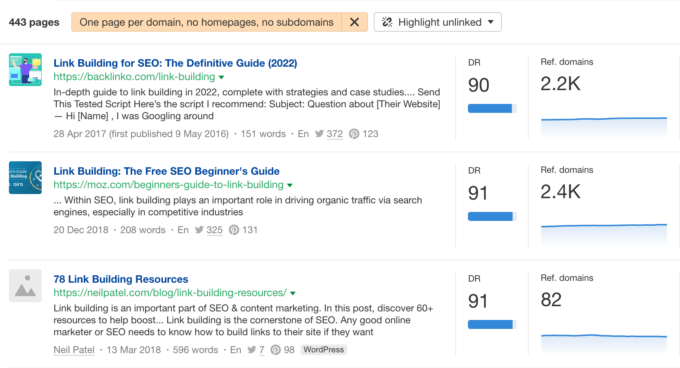This image is a screenshot displaying search results related to link building for SEO. The top-left corner of the screenshot shows the text "443 pages" in black. Adjacent to this text, a tan-colored rectangular notification box indicates a filter with the criteria: "one page per domain, no homepages, no subdomains." To the right of this box is a dropdown menu labeled "highlight unlinked," suggesting there are additional options available.

Below this section, three articles are listed. The first article is titled "Link Building for SEO: The Definitive Guide 2022." To its right, it displays a Domain Rating (DR) of 90 and a reference domain count of 2,200.

The second article is titled "Link Building: The Free SEO Beginner's Guide." This article boasts a DR of 91 and a reference domain count of 2,400.

The final article, "78 Link Building Resources," features a DR of 91 but significantly fewer reference domains, totaling 82.

Each article entry provides valuable metrics related to their domain rating and the number of reference domains, emphasizing the comparative strength and reach of each resource.